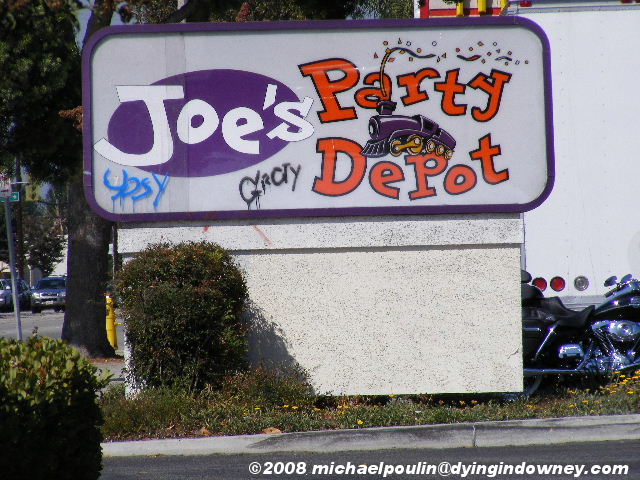The image captures a landscape-style scene featuring a sign that reads "Joe's Party Depot." The sign, situated on a white stucco-finished, gray stone base, sports a thin purple outline, with a light purple interior. "Joe's" is prominently displayed in white text on a purple oval on the left half of the sign, while "Party Depot" is written in bold orange letters, with a small purple train nestled between "Party" and "Depot" on the right half of the sign. Graffiti, consisting of blue and black spray-painted words, can be seen under the letters "J" and "S" in "Joe's." The foreground features a green grassy area with yellow daisies or dandelions, and a tall green bush stretches up to the bottom left of the sign. A black and silver motorcycle is partly visible behind the sign, along with a portion of a truck. To the left, a tree emerges from the sidewalk, accompanied by two cars on the street and a yellow fire hydrant. The very bottom of the image includes the white text: "copyright 2008 Michael Poulin at dyingindowney.com."